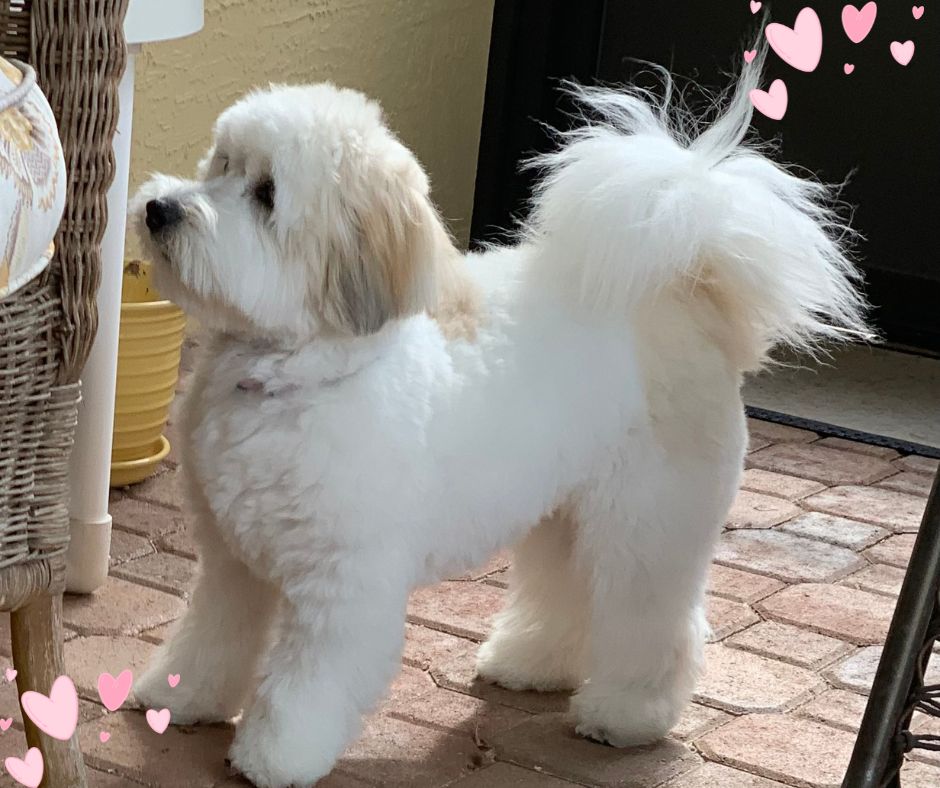In this photograph, a well-groomed, white fluffy dog with faint light brown patches on its tail end and back stands on a meticulously arranged pattern of brick pavers in a backyard setting. The medium-sized dog, aged approximately 3 to 6 years, is poised on all four feet, looking slightly upwards towards a wicker chair situated near it. The scene is bathed in sunlight, accentuating the dog's clean, poofy coat. Behind the dog, there's a flower pot and a yellow wall to the side, with a black surface displaying pink hearts just above its tail. Additionally, digital pink heart designs have been added to the bottom left and top right corners of the image, enhancing its visual appeal. This charming outdoor snapshot captures a moment of curiosity and well-being in the pet's environment.